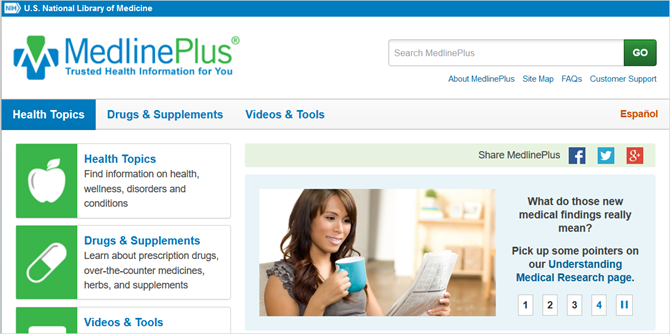**Screenshot of U.S. National Library of Medicine Website Interface**

The image features a detailed screenshot of the U.S. National Library of Medicine's website interface. Positioned prominently is a tiny, white logo that appears to resemble a tag, directing attention to the "U.S. National Library of Medicine" title.

Below the main header, the "MedlinePlus" logo is displayed, which includes a distinctive cross design—half blue and half green—with an "M"-shaped graph within the cross. The text "Medline" is in blue, while "Plus" is in green, featuring a capital "P" and the word "Plus." Beneath the logo sits the slogan, "Trusted Health Information for You."

To the right of the logo is a functional search bar labeled "Search MedlinePlus," accompanied by a Go button for submitting queries.

Below the search section are several navigation links in blue, including "About MedlinePlus," "Sitemap," "FAQs," and "Customer Support."

The main menu is clearly visible, with the "Health Topics" category highlighted in blue, indicating the current selection. Other menu options visible include "Drugs and Supplements" and "Videos & Tools." To the far right of the menu is an option for Español.

The primary content area is sectioned into different boxes:
- One box labeled "Health Topics."
- Another labeled "Drugs & Supplements."
- A third labeled "Videos & Tools."

Adjacent to these sections is a feature for sharing MedlinePlus content.

At the bottom right, a section delves into interpreting new medical findings, offering users pointers on various topics, listed numerically from one to four. A pause button is also displayed, likely related to a video or interactive element within the page.